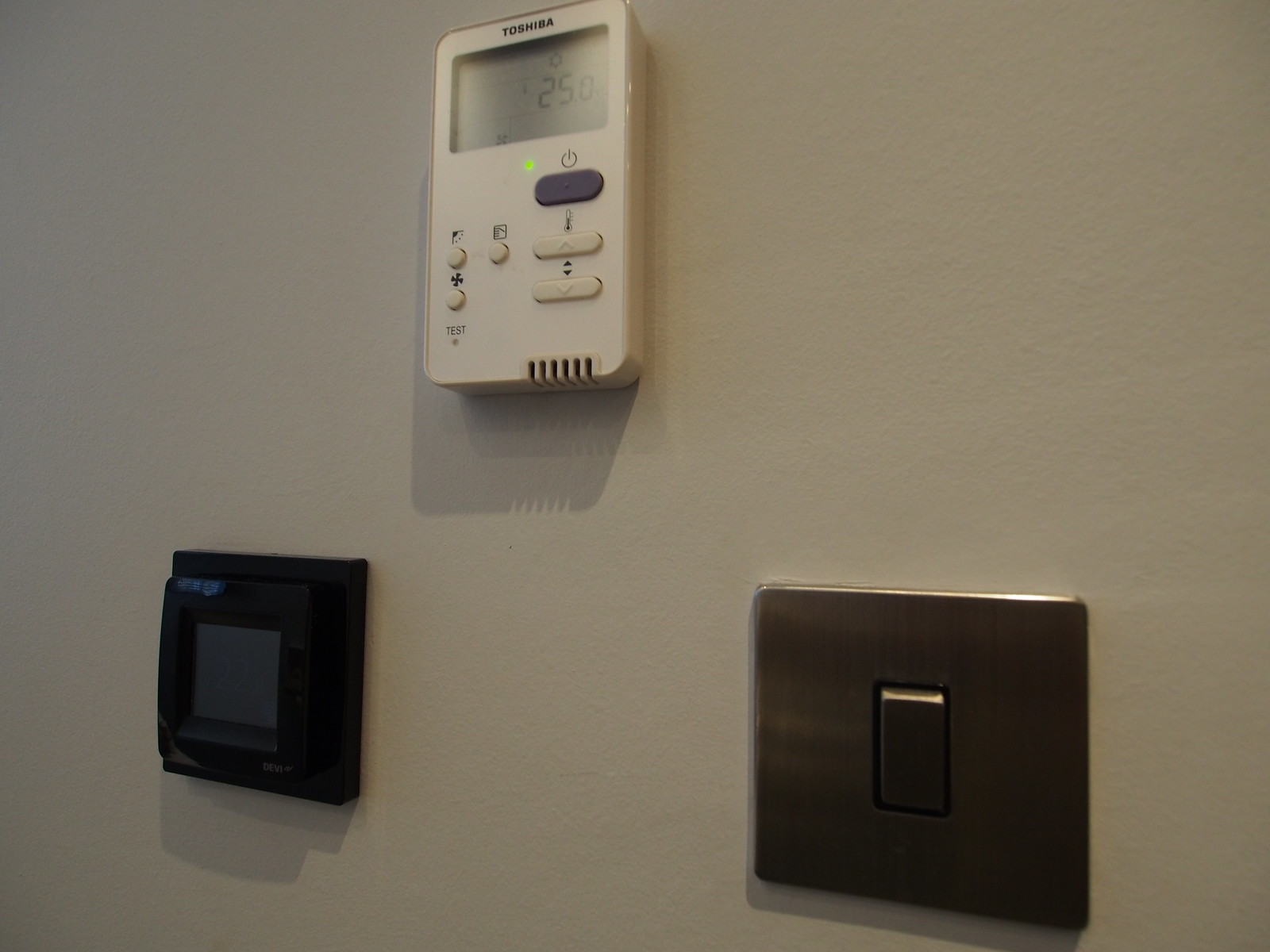This photograph features a modest section of an off-gray wall with three distinct items affixed to its surface. Dominating the upper part of the image, slightly centered, is a Toshiba white thermostat displaying a temperature of 25 degrees Celsius, indicative of a non-American setting. The thermostat, characterized by its old-fashioned gray and black digital interface, includes several functional elements such as a power button located beneath the display, along with temperature adjustment arrows and additional buttons, including a test button.

Beneath the thermostat are two more fixtures. The first is an enigmatic black square device that appears electronic, though its purpose isn’t immediately clear as the potential screen on it is currently dark. Below this device is a metallic-bronze plate housing a sufficiently large light switch. The combination of these elements against the plain wall offers a glimpse into the various utilities integrated into this particular space.